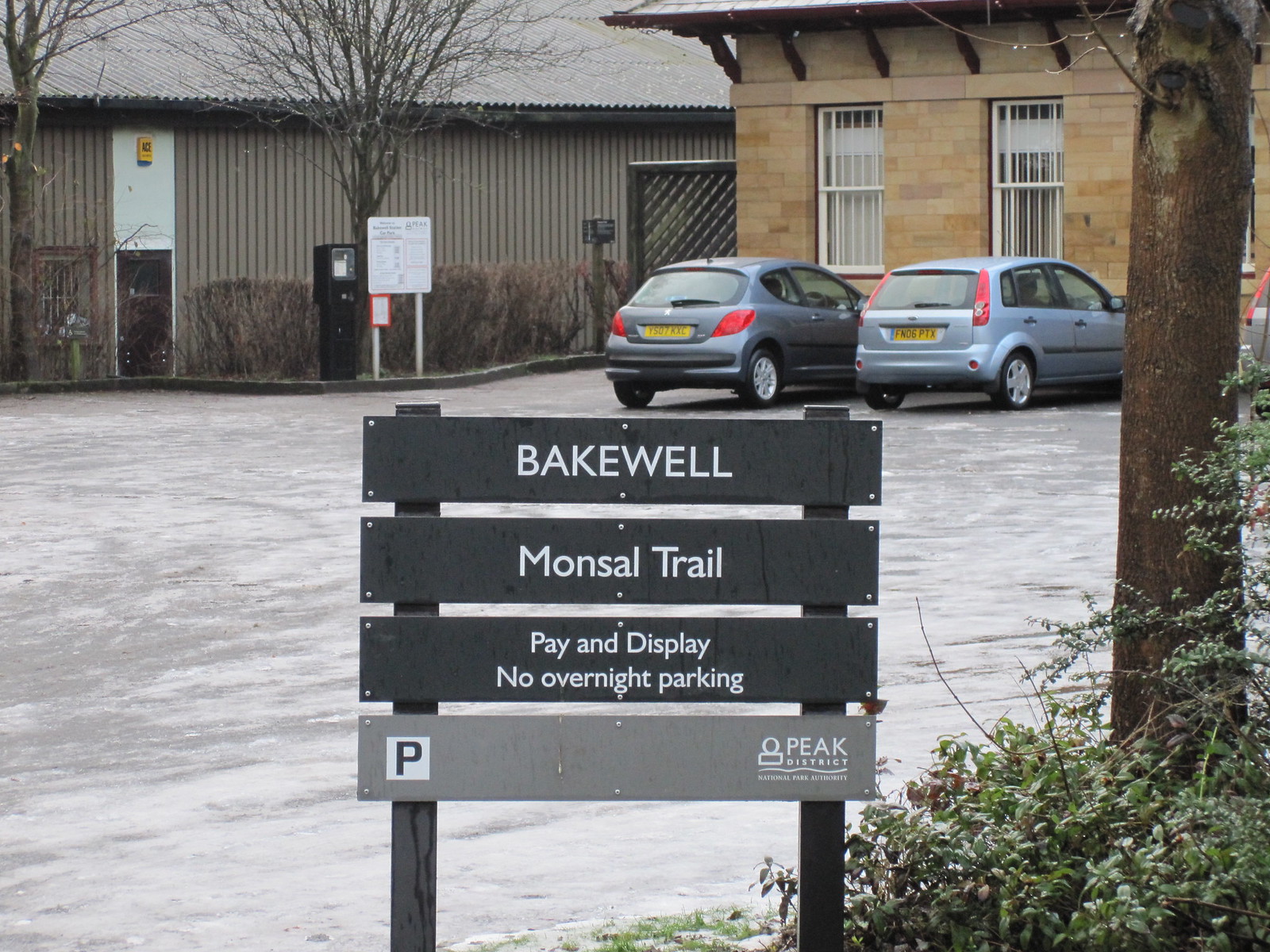The photograph captures a parking lot on a seemingly wet day, possibly following rain, with a prominent sign in the foreground and some buildings in the background. The sign consists of four horizontally stacked panels, supported by two square-shaped signposts on either side. The top three panels are black with white text and read, from top to bottom: "Bakewell," "Monsel Trail," and "Pay and Display. No overnight parking." The bottom panel is light gray, featuring a white square with a black letter "P" on the left side and "Peak District" in white text on the right. Adjacent to the sign, on the right, stands a brown tree with multiple bare branches and a green bush at its base. The parking lot appears icy, amplifying the sense of recent wet weather.